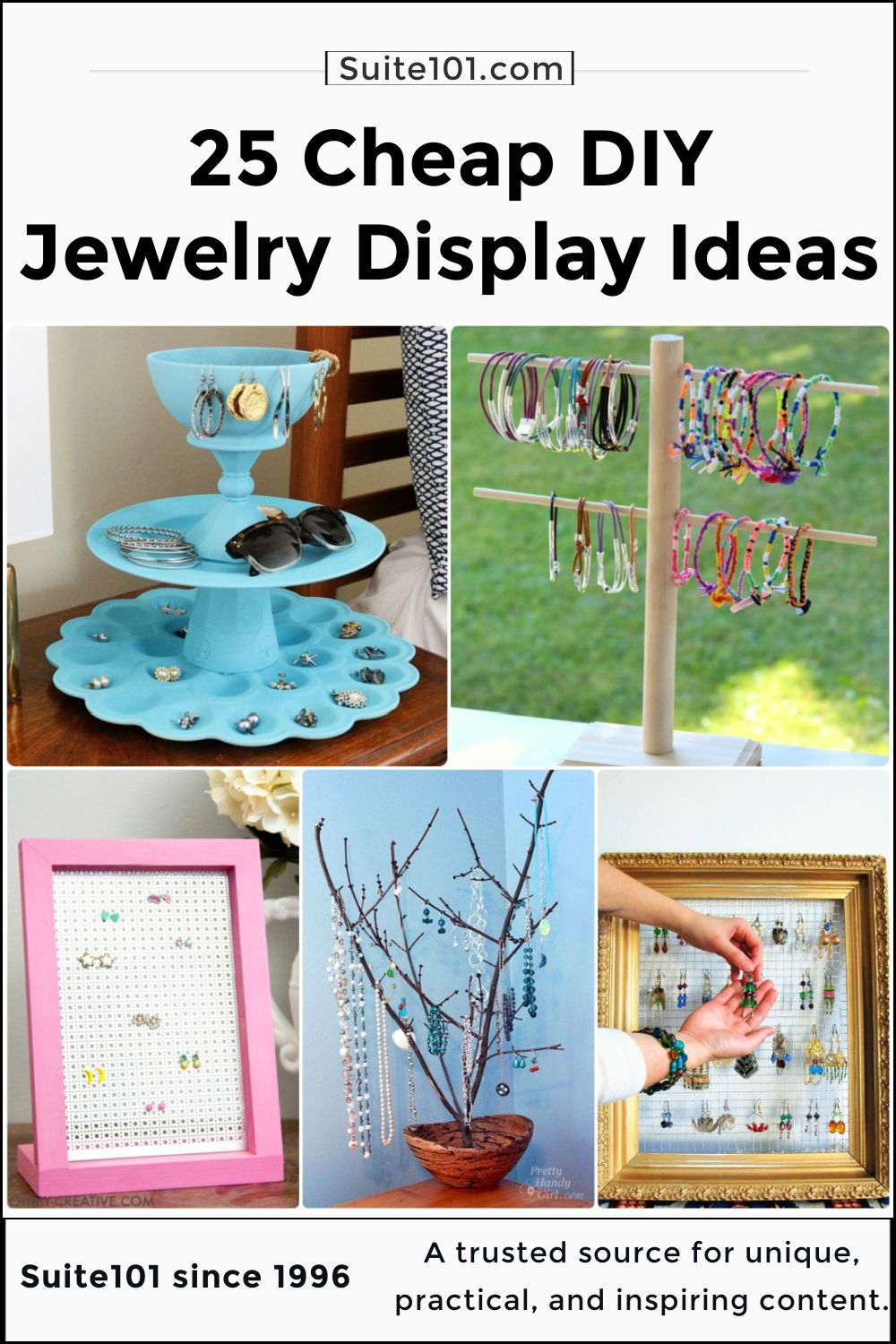The image, likely the cover of an advertisement or flyer for Do-It-Yourself Jewelry Displays, features a predominantly white background enclosed by a thin black border. At the top, in small lettering within a black box flanked by thin blue lines, is the text "Sweet101.com." Beneath this is bold black writing proclaiming, "25 Cheap DIY Jewelry Display Ideas." Surrounding the title are various images showcasing creative jewelry display solutions:

- A multi-layered display starting with a bowl atop a plate, which in turn rests on an egg dish. Sunglasses and earrings adorn different layers, with the earrings hanging over the edge or placed within the egg compartments.
- A small wooden stand resembling a bird perch with two layers of rods, each end supporting numerous bracelets.
- A pink frame used to hold and display earrings.
- A basket with tree branches extending upward, creatively supporting earrings and other jewelry.
- A gold frame also utilized to showcase various jewelry pieces.

At the bottom of the image, it states, "Sweet 101 since 1996," affirming itself as "a trusted source for unique, practical, and inspiring content."